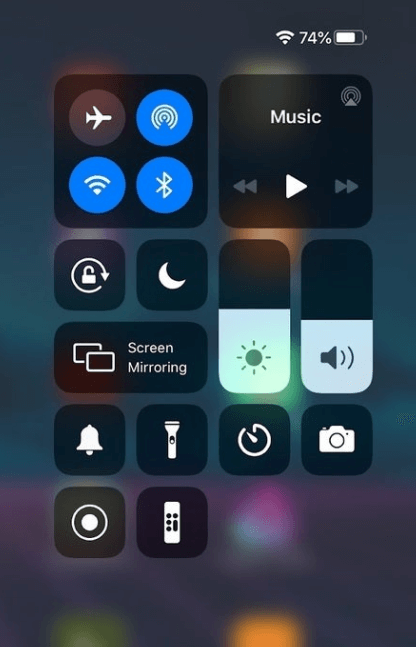This image showcases a close-up of an iPhone screen displaying the Control Center, set against a blurred background. The Control Center is divided into several sections, each containing multiple icons and functions that are essential for managing the phone's settings quickly.

On the far left, there's a module with four circular icons arranged in a grid. The top-left icon, representing Airplane Mode, is in blue, indicating that it is active. Below it, a blue icon shows the status of the Wi-Fi network, with another blue icon below this representing Bluetooth. The top-right icon is gray, indicating signal network status.

To the right of this section, another box labeled "Music" displays media controls. The play button is flanked by rewind and reverse buttons, allowing you to navigate through your music.

Below these sections, centrally located, is a lock icon representing the screen orientation lock, next to a circular icon depicting a moon, which signifies the Do Not Disturb mode.

Further down, a rectangular box indicates the Screen Mirroring feature, used to project the iPhone's screen onto other devices.

Lastly, at the bottom, there are two more controls: a rectangle with a sun icon used for adjusting screen brightness, and a speaker icon for volume control.

In summary, this image provides a detailed view of an iPhone's Control Center, highlighting the various settings and controls available for quick access on the device.